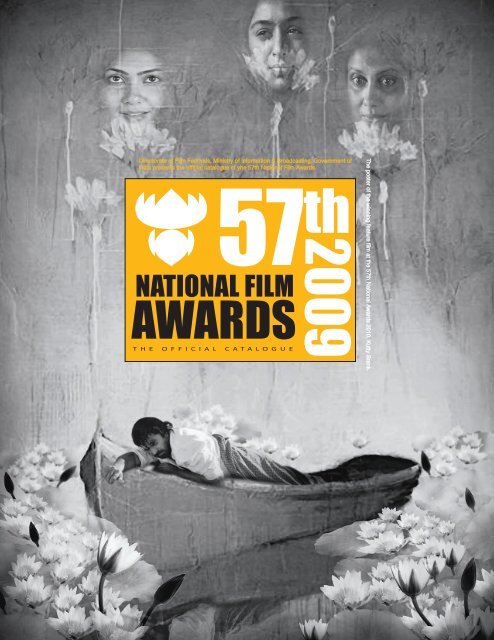The image appears to be an advertisement for the 57th National Film Awards held in 2009, prominently showcasing the official catalog. The primary visual consists of a black and white background, enhancing its artistic appeal. At the bottom, there is a man with dark hair and a beard, looking pensively at the water from an open boat or canoe, surrounded by what appear to be white flowers on either side. In the center of the image, an orange box with white and black text reads "57th 2009 National Film Awards, the official catalog." Above this box are the ethereal faces of three women, each adorned with flowers beneath their faces against a gray backdrop. In the top left corner, a small logo or symbol, possibly depicting a stylized crown or head with large ears, is barely discernible due to its abstract design.